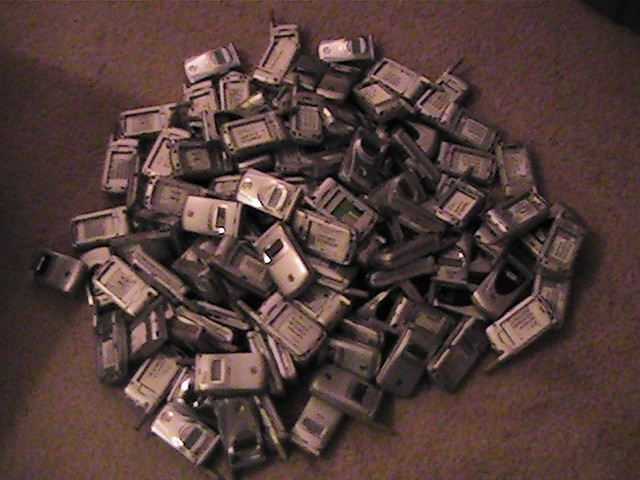The image is an overhead photograph of a large pile of old silver flip cell phones on a grainy gray-beige surface, possibly a carpeted floor. The image is slightly blurry, and there are shadows visible on the left side and a dark corner in the top right. Most of the flip phones feature dark gray antennas and have removable battery compartments, all of which appear empty, indicating the batteries are missing. The cell phones display rectangular LCD screens on their fronts, and the variety of makes and models suggest multiple brands. Some phones are flipped open, revealing their interiors, while others are closed. A few phones appear broken, showing only halves of the devices. The phones are stacked several layers high, creating a large, disordered pile.